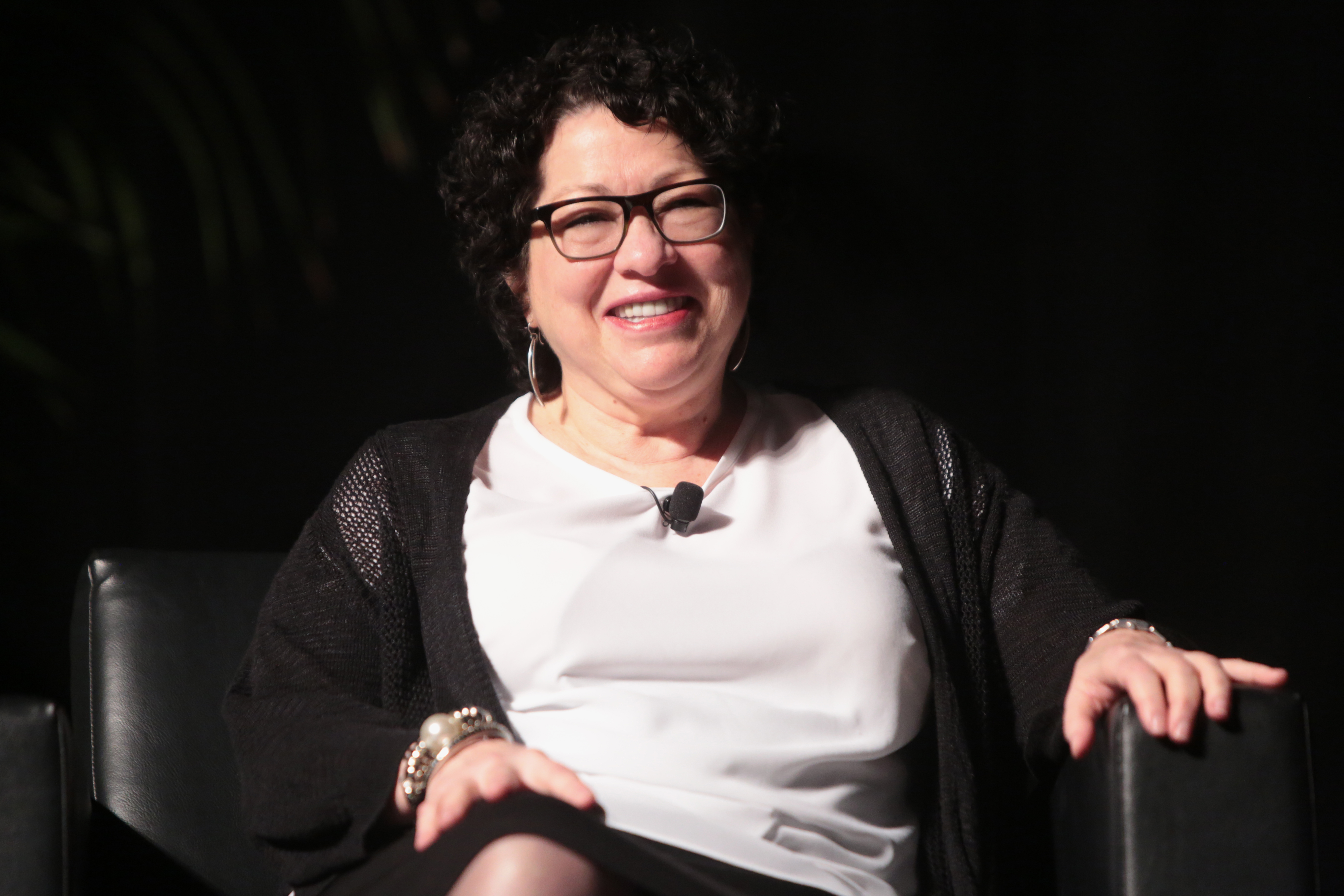This detailed image captures Supreme Court Justice Sonia Sotomayor, who appears to be seated in a short-backed black leather chair. She is dressed in a thin-knit style black jacket over a white t-shirt, with what seems to be a black skirt, though the exact details are hard to discern. Justice Sotomayor is wearing thick black glasses and has dark curly hair cut to about shoulder length. She smiles softly, with a slight squint in her eyes, suggesting she is looking at an audience in front of her.

A small black microphone is clipped to the center of her shirt, indicating she may be engaged in a speaking event. On her left wrist, she sports a gold or silver wristwatch, while her right wrist is adorned with a couple of golden or silver bejeweled bangles, one of which might feature a pearl. Her right hand rests on her right knee. Additionally, she is wearing large silver earrings.

The backdrop is very dark, perhaps with a subtly wavy texture that hints at a curtain, yet offers no further contextual clues about the location. The overall atmosphere and elements in the image contribute to a focused and possibly formal setting.